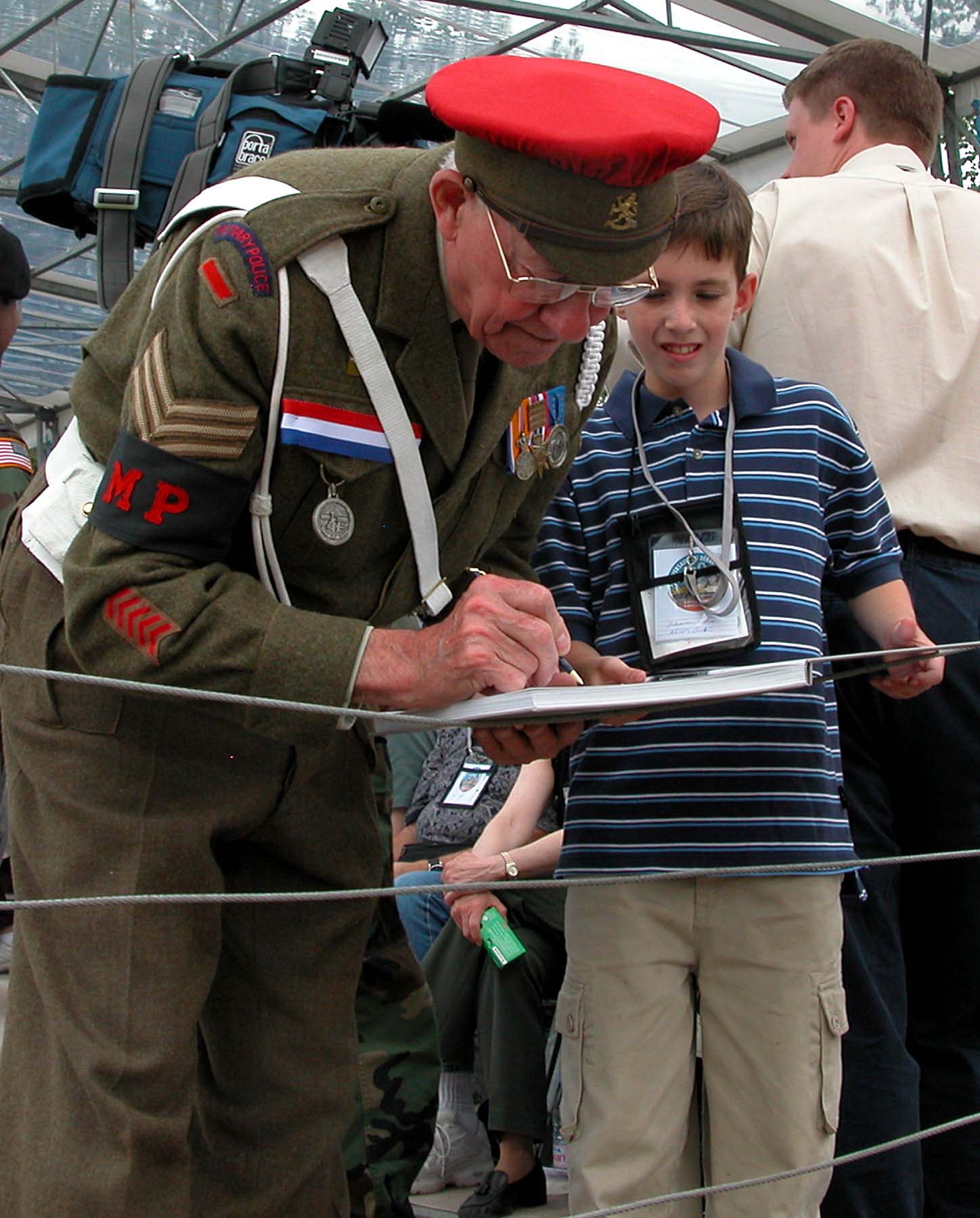In this vibrant photograph, an elderly veteran, likely in his 80s, is dressed in a distinct, colorful military uniform of greenish-brown, adorned with medals and patches. Notably, a red boating cap with a brown underside sits atop his head, and a black armband with the letters "MP" in red is wrapped around his sleeve, which also bears a sergeant's stripe. The veteran wears glasses and is engaged in signing something for a young boy, who appears to be around 8 to 10 years old. The boy is dressed in a navy blue polo shirt with light blue and white stripes, along with khaki cargo pants. They are leaning over a barricade made of wire string, possibly indicating a structured or event setting. In the background, there are people, a TV camera, a building, and various objects including water bottles and ID tags, hinting at a formal gathering or commemorative event. The scene is illuminated with colors of red, blue, white, green, tan, and black, and both the veteran and the boy are facing the camera, capturing a moment of interaction and reverence.